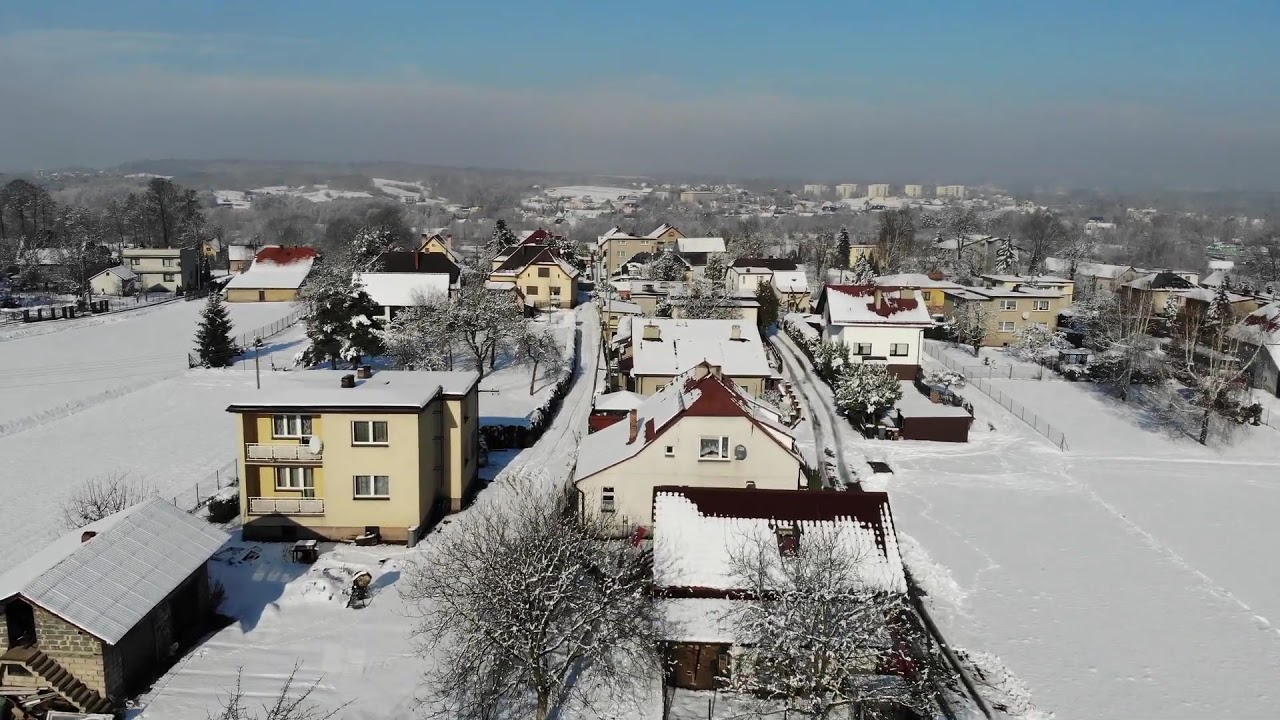The image depicts an aerial view of a small, wintry residential area taken from a drone. Below, you see a scattering of dated houses and small apartment buildings, each with cream-colored walls and red clay rooftops covered in a fresh blanket of snow. The snow blankets the entire landscape, from the roofs of the houses to the ground and trees. The homes are spaced out, with some featuring balconies, and there's a mix of open areas around them. In the foreground, a few houses are prominently positioned, leading towards additional houses and small buildings that stretch horizontally behind them. In the background, hills and clusters of trees envelop the town, and further out, larger buildings can be spotted. The sky is overcast, with patches of blue visible above the clouds, emphasizing the quiet, wintry atmosphere of this serene small town.